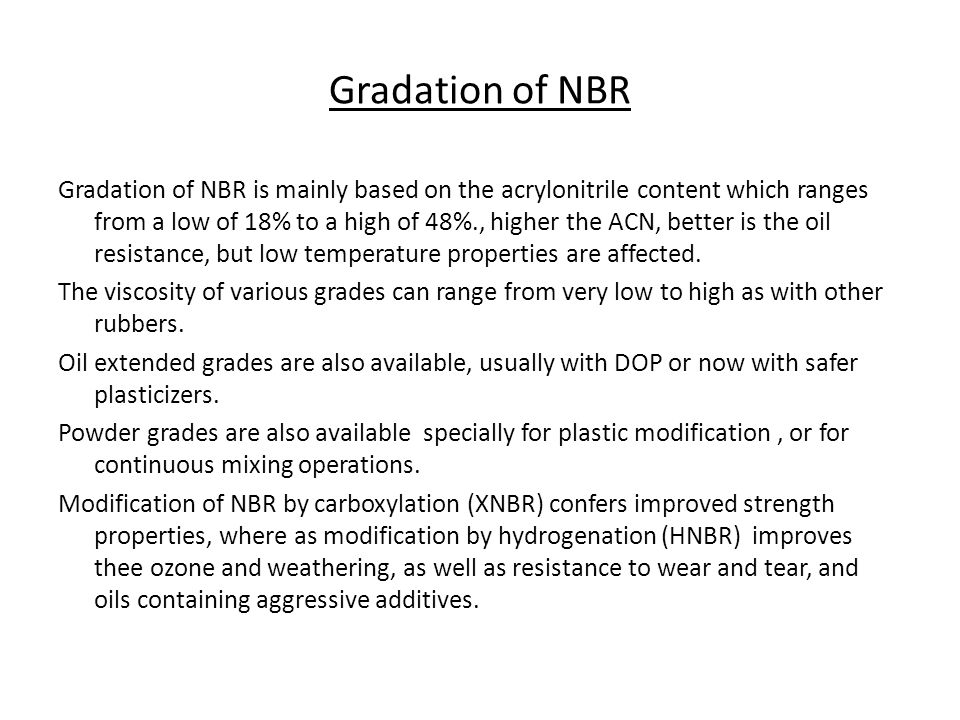The image presents detailed information about the gradation of NBR (Nitrile Butadiene Rubber), displayed on a white background with black text. A prominent, underlined title reads "Gradation of NBR," followed by a comprehensive explanation in smaller print. The gradation of NBR is primarily based on its acrylonitrile (ACN) content, which varies from 18% to 48%. A higher ACN content improves oil resistance but negatively impacts low temperature properties. The viscosity of the NBR grades spans from very low to high, comparable to other rubbers. Some grades are oil-extended, typically with DOP, though safer plasticizers are now also used. Additionally, powder grades are available for plastic modification or continuous mixing operations. Carboxylating NBR enhances its strength properties, while hydrogenating NBR (HNBR) increases resistance to ozone, weathering, wear, tear, and aggressive additives in oils.